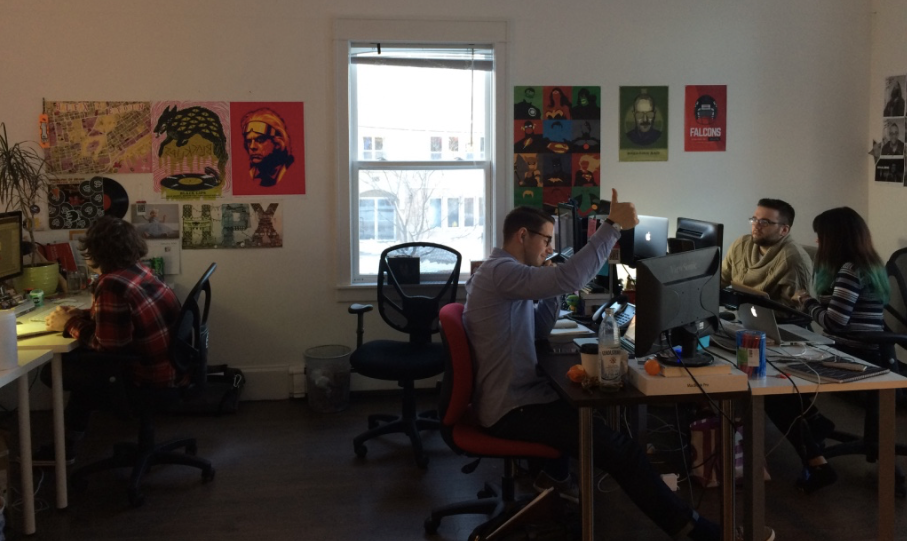The image depicts a lively, indoor scene set within a well-lit office room or classroom featuring a diverse group of individuals engaged in various activities. The room has wooden floors and white walls adorned with various posters and pictures. A large window with open shades reveals another building outside. On the left side of the image, a man with dark hair, wearing a black and red plaid shirt, is intently looking at a computer screen, illuminated by its light. Above his desk, there's a plant, adding a touch of greenery to the room.

Towards the center, a man with short dark hair, a beard, and glasses, dons a long-sleeve blue shirt while sitting in a red chair. He is energetically giving a thumbs-up with one arm raised. In front of him, the desk is scattered with items including a bottle, a cup, and an orange. The workspace also features several computer monitors. To the right, a woman and another man, who are both focused on their computer screens, share the desk with him. The woman, identifiable from her back, sports a gray and black-and-white striped long-sleeve shirt with short dark hair, while the man has a greenish shirt and short dark hair.

In the background, yet another individual in a flannel shirt is seen with their back to the camera, also working at a desk. The chairs in the room are varied, some red and others black. A trash can is visible under the window, emphasizing the functional aspects of the space. The overall atmosphere inferred from the image is that of a collaborative setting, filled with engagement and activity, whether it be a classroom, office, or other professional environment.